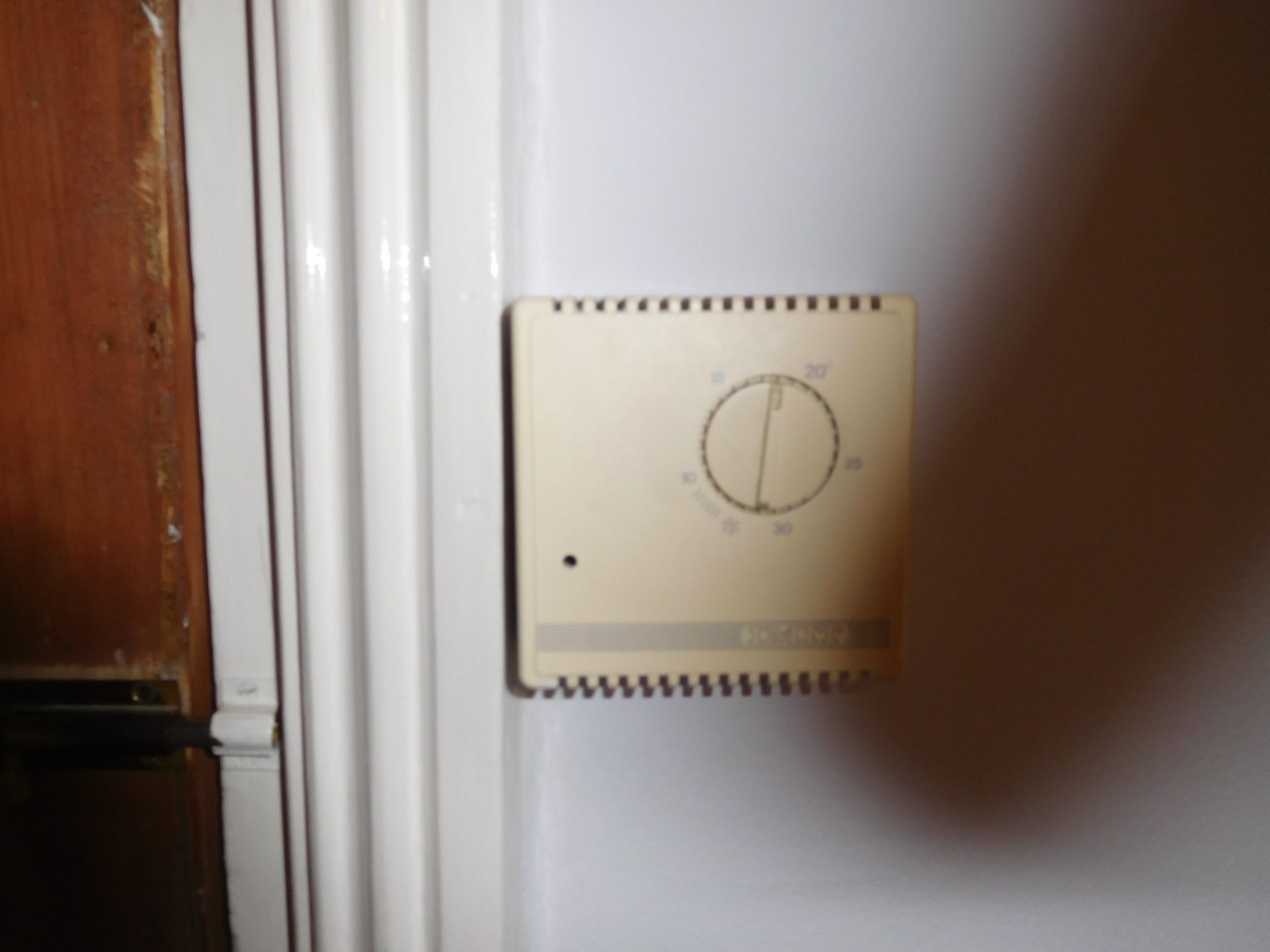This indoor, close-up color photograph captures a square plastic thermostat mounted on a white wall. To the left of the thermostat, the glossy white trim of a door is visible, alongside a portion of the wooden door itself, which is a dark orangish-red hue. The lower center and left edge feature part of a dark metal deadbolt, with a corresponding latch on the white-painted trim. The focal point of the image, the thermostat, is positioned just right of center. It includes vent slots on both its top and bottom edges. 

In the upper right corner of the thermostat, a round dial is present, marked with degree numbers. "20" is discernible, followed by "30" to the right; the rest of the numerals are illegible. The dial has an indicator pointing almost straight up but slightly towards the right. A noticeable dark oval shadow intrudes from the upper right corner, casting across the lower right section of the thermostat. The photograph is poorly lit, slightly grainy, and out of focus, adding a certain texture to the scene.